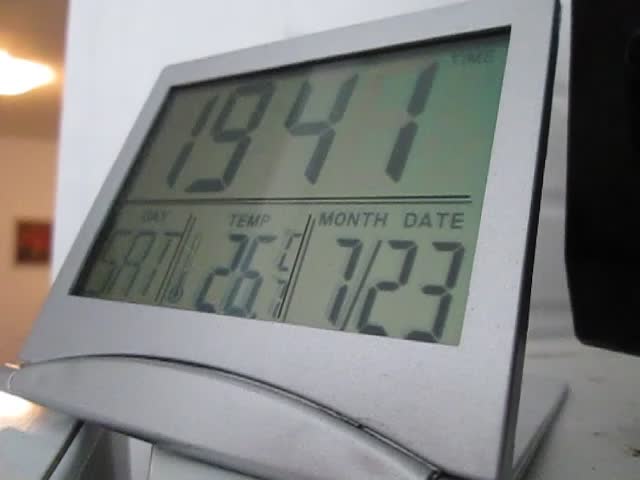This image features a silver, square digital clock displaying military time. The clock, propped at an angle by a bottom flap extending from the back, prominently shows "1941" in digital numbers, indicating the time in hours and minutes. Beneath the time display, two thin black lines separate different informational sections. On the left, the word "DAY" with "SAT" below it signifies that it is Saturday. Adjacent to this, a section labeled "TEMP" shows the current temperature as "26°C." To the right, under the heading "MONTH DATE," the display reads "7/23." The digital numbers stand out against a light green background. The clock rests on a white table, with a portion of it hanging off the edge.